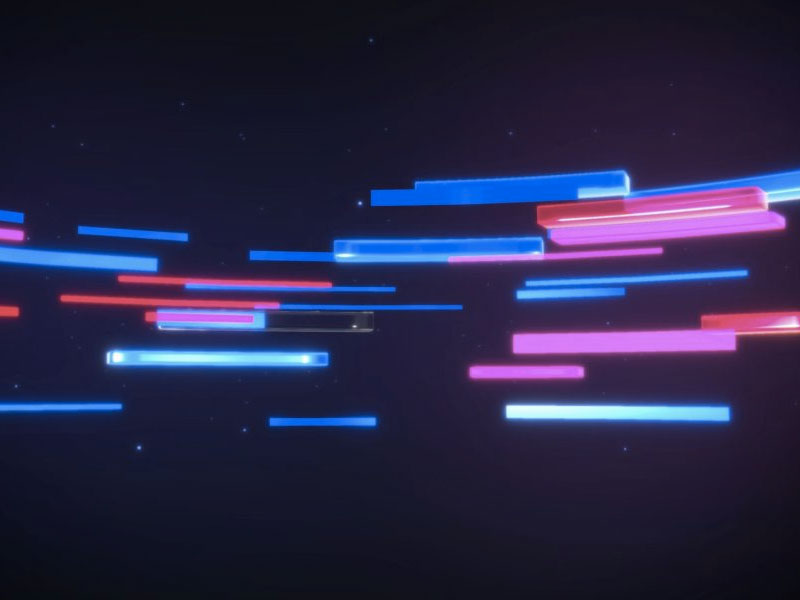The image features a striking piece of light-based artwork set against a solid black background. At its top, a light blue streak with a notch cut out on the left side begins the composition. Descending from the top right, there's a lighter blue patch, followed by a darker pink streak adorned with a white line, and beneath that, a light purple streak. These streaks are slightly curved at their centers, creating a dynamic flow outwards as they widen towards the edges. Across the bottom portion of the image, three almost neatly aligned horizontal streaks appear—each a variation of blue, from light to a bit darker, with the rightmost one being the lighter blue. Interspersed among these streaks are small, glowy white dots that resemble stars. The neon lights, consisting of blue, pink, and hints of red, glow vibrantly, occasionally giving a 3D illusion. The composition of neon light bars is mostly centralized, leaving the edges dark and empty, enhancing the dramatic contrast and depth of the artwork.